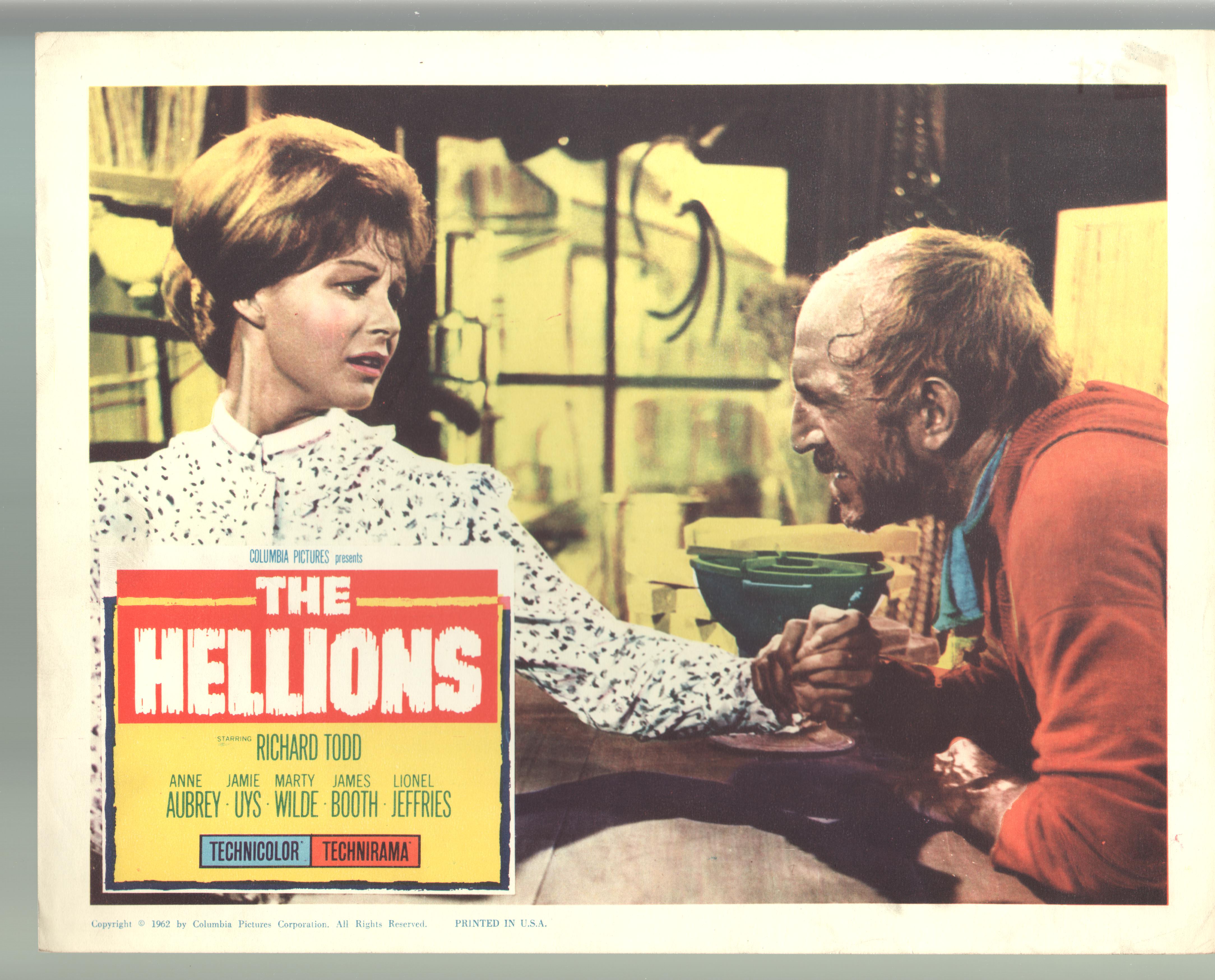This vintage movie poster advertises the film "The Hellions" presented by Columbia Pictures, starring Richard Todd, Anne Aubrey, Jamie Uys, Marty Wilde, James Booth, and Lionel Jeffries. The movie is showcased in Technicolor and Technirama. Dominated by a vivid and distinctive yellow background with green lettering, the poster features a logo in the bottom left-hand corner reading "The Hellions" in white text against a red backdrop. The names of the stars, Technicolor's text in blue, and Technirama's text in red enhance the vintage aesthetic.

The poster includes a still from the movie: a woman and a man are depicted inside an old house. The man, appearing distraught in a red shirt, is holding the woman's hand—seemingly entreating her with some urgent or bad news. The woman, dressed in a white shirt, looks at him with warm, sympathetic eyes. The backdrop outside the house is notably yellow, further adding to the overall vintage tone of the scene. The poster is surrounded by a white frame, enhancing its classic, framed-photo appearance. Printed in the USA.